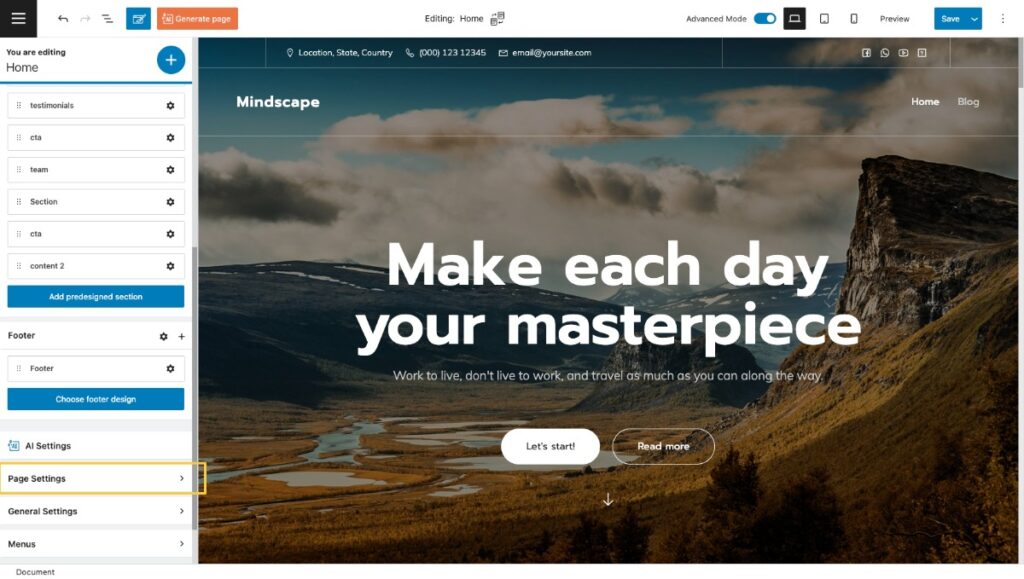A detailed screenshot of a website builder interface is shown. This interface, either a web application or software, features multiple tools and settings, though the taskbar and search navigation bar are not visible. On the bottom left, there is a highlighted button labeled "Page Settings," suggesting it's part of an infographic or tutorial. 

In the top left corner, a hamburger menu button is positioned next to various operational buttons including undo, formatting options, edit, and an orange button with text options. The top bar also comprises a selector for different device formats—desktop, tablet, and mobile—followed by buttons for "Previous," "Save," and a three-dot menu. The text "You are editing home" indicates that the homepage is currently being edited.

The homepage design features a full-screen image of a plateau and mountainous region bathed in dawn light, with a golden, plains-like appearance and a cloudy sky. Overlaid on this image at the top are fields for a location, state, country, phone number, and email, none of which are filled in. The website is titled "Mindscape" and includes navigation buttons for "Home" and "Blog."

Inspirational text graces the homepage: "Make each day your masterpiece. Work to live, don't live to work, and travel as much as you can along the way." A button labeled "Let's start" and a "Read More" link provide additional interaction points. To the left, a sidebar menu likely facilitates navigation through sub-sites or sub-pages within the website.